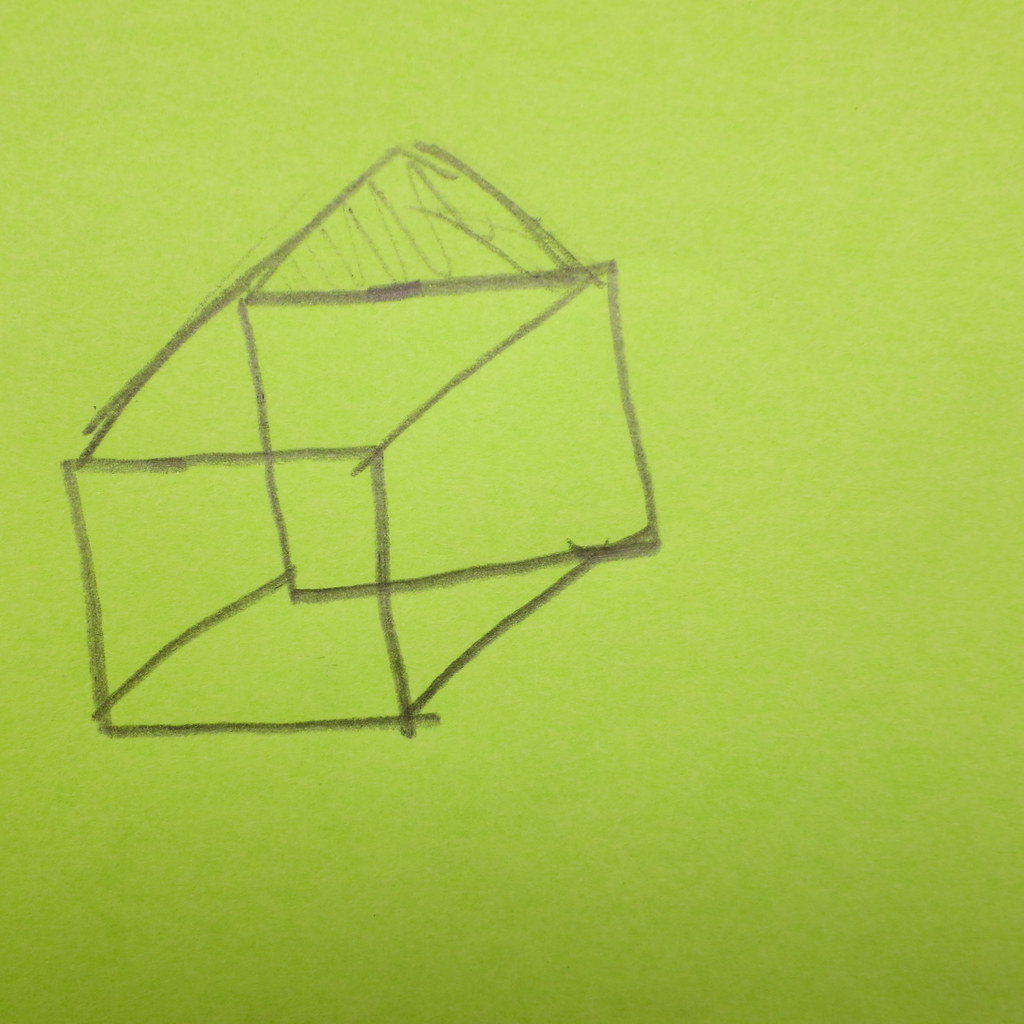This simple sketch features a basic, three-dimensional box rendered in precise line art with graphite on chartreuse green paper, resembling a large Post-it note. The drawing predominantly showcases the front and one adjacent side of the box, with lines and angles suggesting depth and perspective, although the far side and back are not visible. Intriguingly, a triangular shape atop the box hints at a roof-like structure, giving it an appearance somewhat reminiscent of a house, though this may not be the artist's intent. The image, likely scanned, maintains a clean and clear rendition of the drawing despite its general lack of contrast and vibrancy, relying instead on the natural brightness of the green paper to add a subtle liveliness to the otherwise minimalist composition.